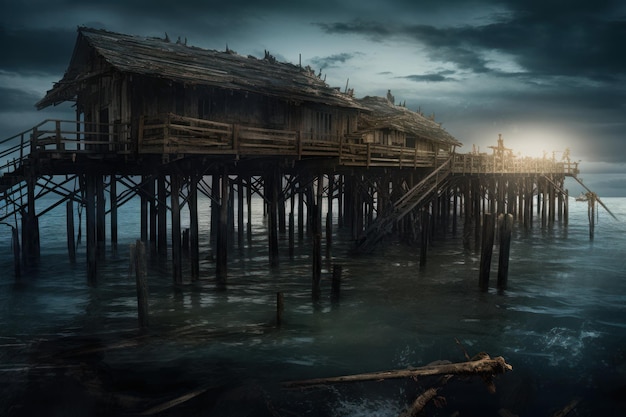The image displays a dark, somewhat ominous scene featuring an old, dilapidated dock extending into the water. The dock, supported by dozens of sturdy wooden pylons, is constructed entirely of wood and has been weathered by time, giving it a gray and run-down appearance. Portions of the dock that were once covered now feature a busted-up roof, with some broken pieces scattered in the water below. Toward the end of the dock, which remains open and extends well into the tranquil gray-blue and white water, a small house or shack rests precariously. The image is horizontally divided, with the lower half depicting the calm, placid water, while the upper half showcases an overcast sky filled with dark clouds. The sky is tinged with the soft hues of either a setting or rising sun, creating a lighter area near the horizon. The sun, a small orb of light, casts a faint glow at the end of the dock, adding to the overall foreboding and melancholic atmosphere of the scene.